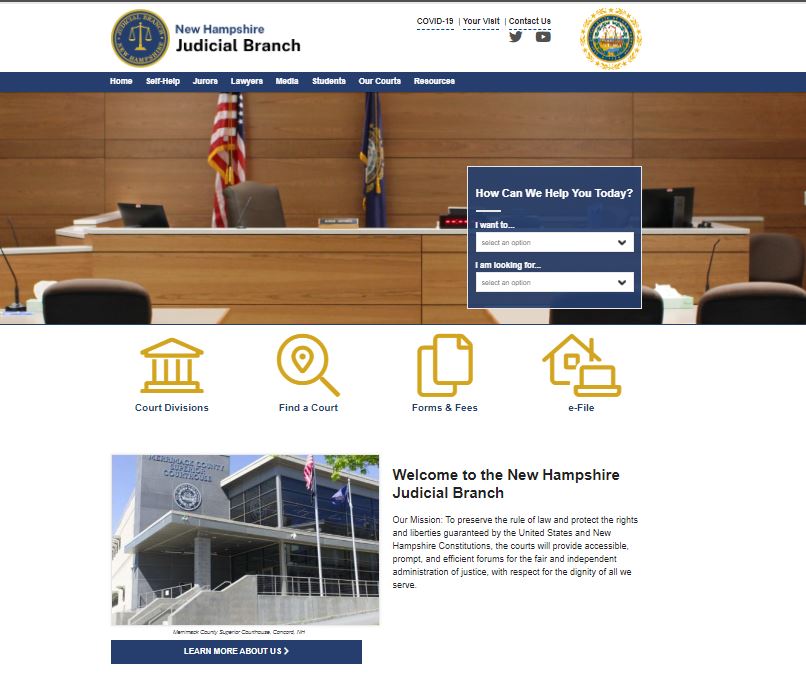The image is a screenshot of the New Hampshire Judicial Branch website. At the top of the page, there is a navigation menu with tabs labeled: Home, Self Help, Jurors, Lawyers, Media, Students, Our Courts, and Resources. Directly below this menu, there are two dropdown menus titled, "How can we help you today?" and "I want to," allowing users to select various options.

Underneath these dropdowns, there are several quick links to key sections: Court Divisions, Find a Court, Forms and Fees, and e-File. Further down, there is a welcoming message from the New Hampshire Judicial Branch detailing their mission to preserve the rule of law and protect the constitutional rights and liberties, providing fair and independent forums for justice while respecting the dignity of those they serve.

Additionally, there is another quick link labeled "Learn More About Us." The website also features a prominent image of a courtroom as the main photo at the top, and an image of the judicial building is displayed further down the page.